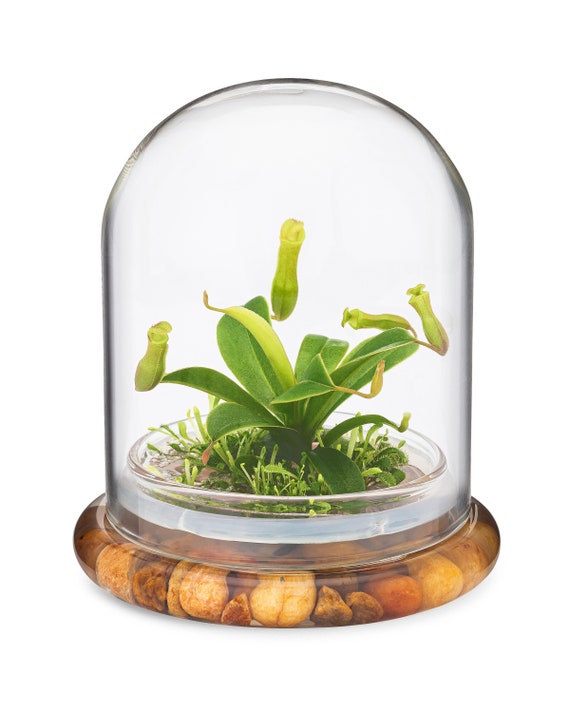The image depicts a decorative terrarium, resembling a small, enclosed growing area situated on what appears to be a flat, circular base. This base, described as having a coaster-like appearance with a lip, is filled with an assortment of yellowish-orange pebbles. There's speculation that the base could be made of clear epoxy or resin embedded with rocks, creating a multi-colored effect with red, white, and brown hues.

Encasing the plant is a curved, glass dome which heightens the appearance reminiscent of a snow globe or even a firmament. Inside, there is a single, prominent plant exhibiting medium green foliage from which delicate, curved branches extend. These branches are adorned with small pods, resembling bell-shaped flower buds, imparting an additional touch of elegance. Around the base of the primary plant, patches of green grass add to the verdant scene.

Some interpret this as a coffee table adornment or a tourist keepsake, questioning whether the plant is real or an artificial creation, possibly made from construction paper. Despite the doubt over its authenticity, the meticulously crafted base with its variety of shades renders it an intriguing and eye-catching ornament.